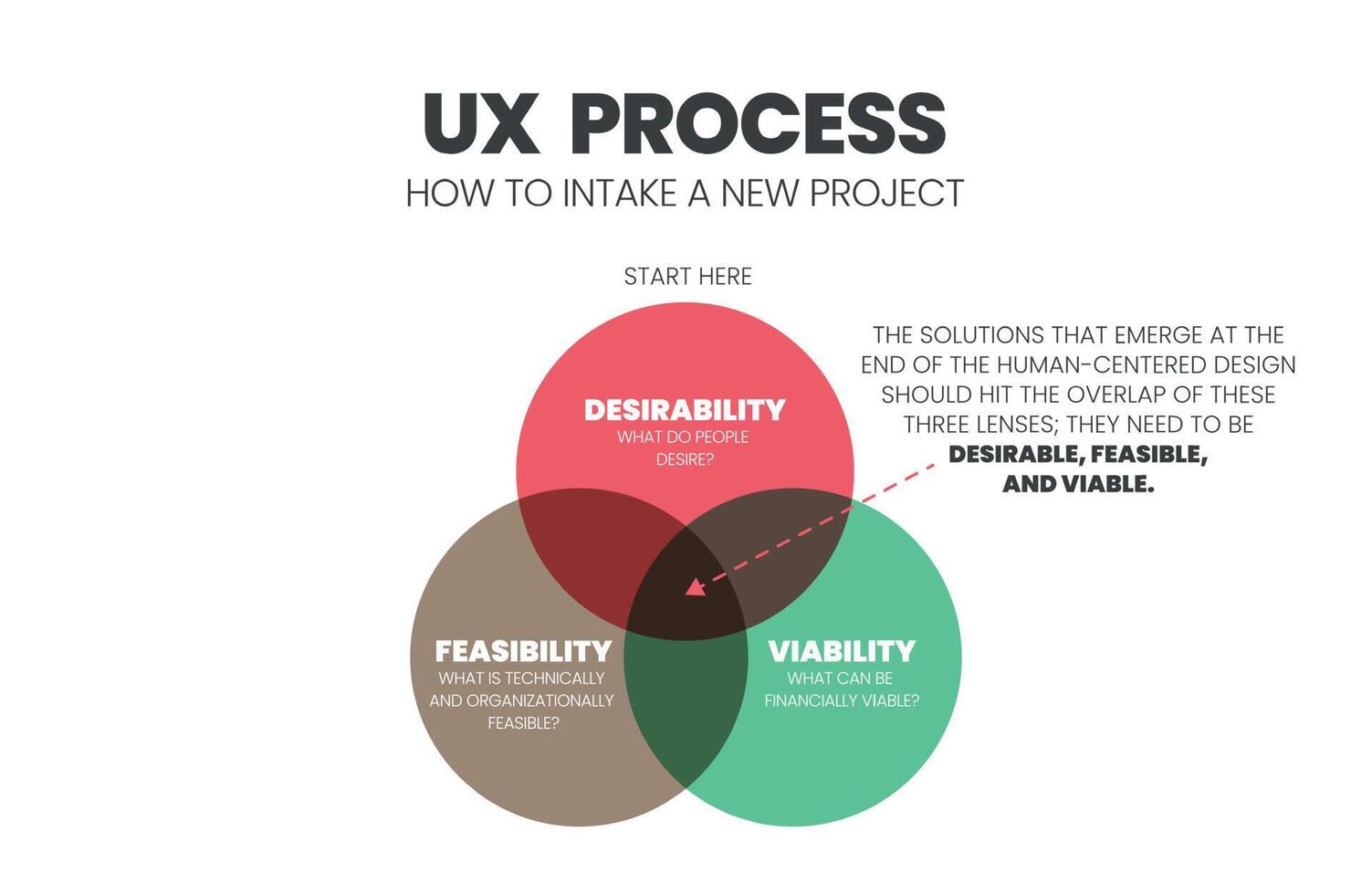The image depicts a detailed flowchart titled "UX Process: How to Intake a New Project" in bold black text. Below the title, in smaller all-caps font, it says "Start Here." The flowchart features three interlocking circles, each labeled with a different key aspect of project assessment. The top circle is red and labeled "Desirability" in bold white text, which addresses the question "What do people desire?" The bottom left circle is brown and labeled "Feasibility," focusing on "What is technically and organizationally feasible." The bottom right circle is green and labeled "Viability," indicating "What can be financially viable." All three circles overlap slightly, converging in the center. A red arrow points to the intersection of these circles, accompanied by the text: "The solutions that emerge at the end of the human-centered design should hit the overlap of these three lenses. They need to be desirable, feasible, and viable." The terms "desirable," "feasible," and "viable" are emphasized in bold font.